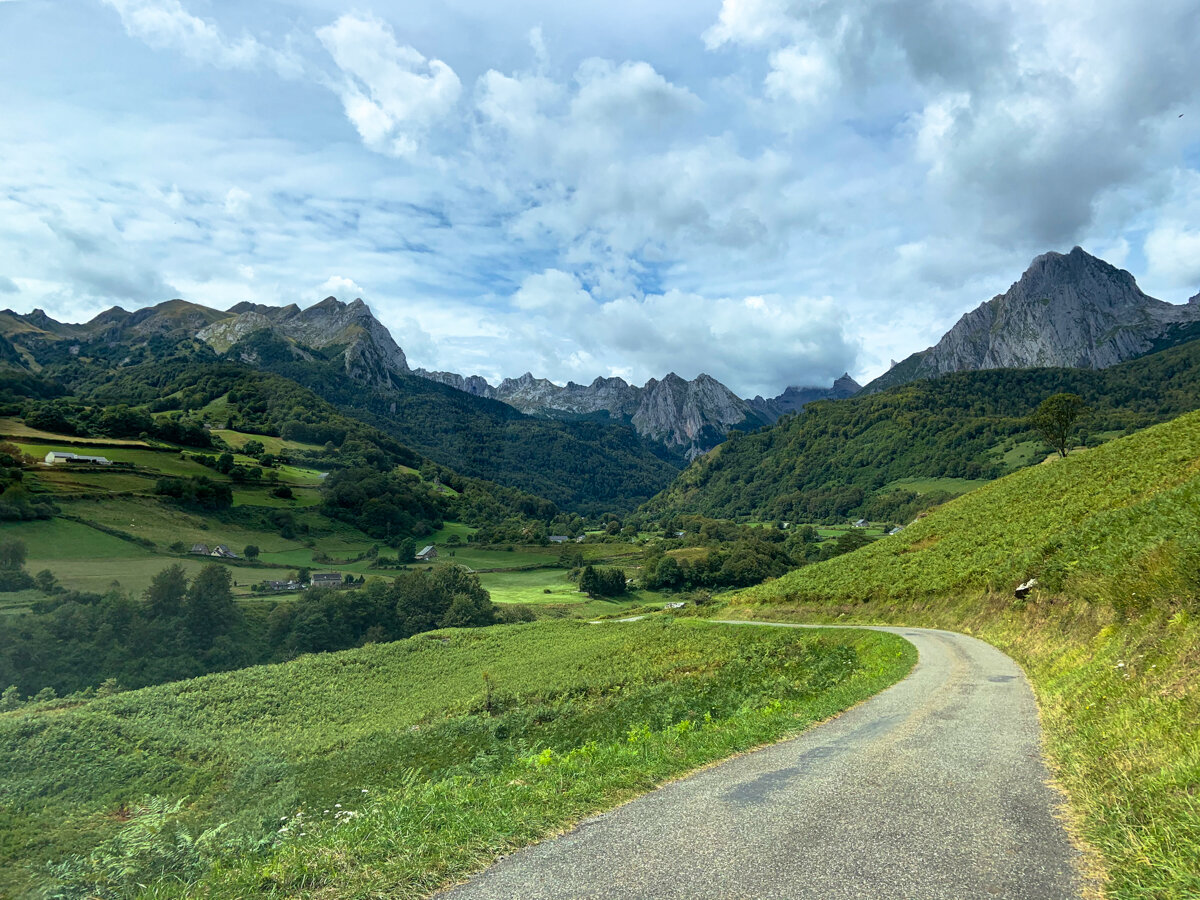This detailed color photograph, taken in landscape orientation, captures a scenic daytime view of Cirque de L'Escoune located in the French countryside. The perspective is from a single-lane concrete walking path that winds its way through the verdant landscape. The path begins at the bottom of the image, curving to the right and disappearing into a lush valley, framed by grassy slopes on both sides. The expansive scene reveals rolling green hills dotted with sparse structures, possibly barns or farmhouses, and stands of dark green trees. In the distance, a dramatic mountain range with sharp, craggy peaks forms the horizon, the highest peak situated to the right. The sky above is a radiant blue, adorned with scattered puffy white and gray clouds, providing a bright yet partially overcast ambiance to the scene. The natural green landscape appears meticulously well-kept, devoid of weeds, and rich in various grasses and shrubs, enhancing the overall picturesque and tranquil atmosphere.